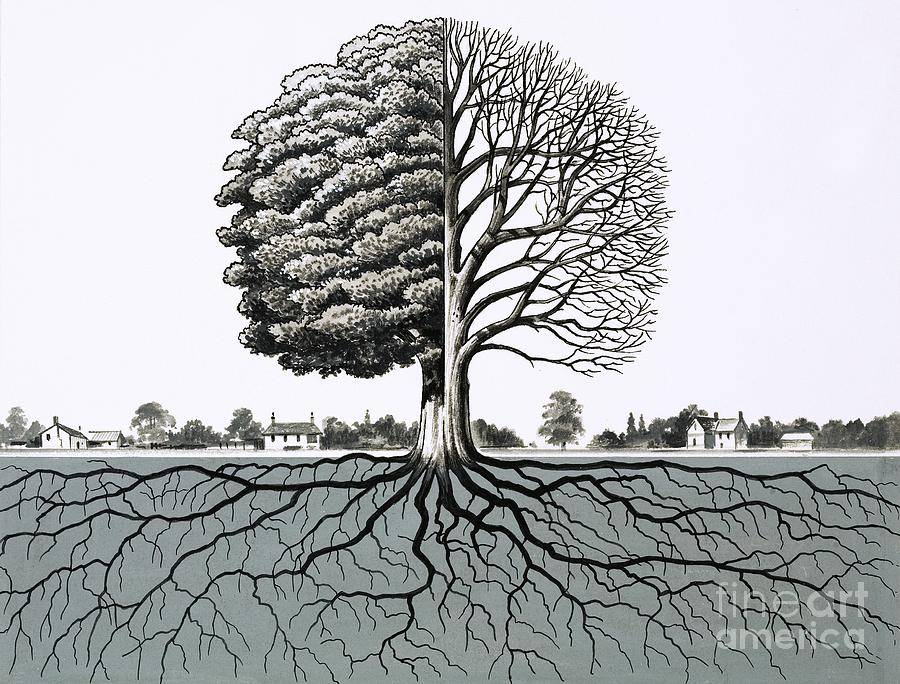In this black and white illustration, a tree stands prominently in the foreground, starkly divided down the middle into two contrasting halves. The left side of the tree is lush and full of foliage, giving off a healthy and vibrant appearance, while the right side is barren, with bare branches that evoke a wintry, sickly feel, devoid of leaves. Despite the drastic difference in the tree's canopy, the roots beneath it are consistently large and dark black on both sides, spreading across the bottom of the image. The background features a subtle outline of a town, with white houses interspersed among other trees, enhancing the serene but divided theme of the artwork. The sky above occupies the top two-thirds of the image, rendered in a plain white shade. In the bottom right-hand corner, the text "Fine Art America" is displayed. This piece captures a stark juxtaposition, emphasizing the contrast between growth and decay, life and dormancy.